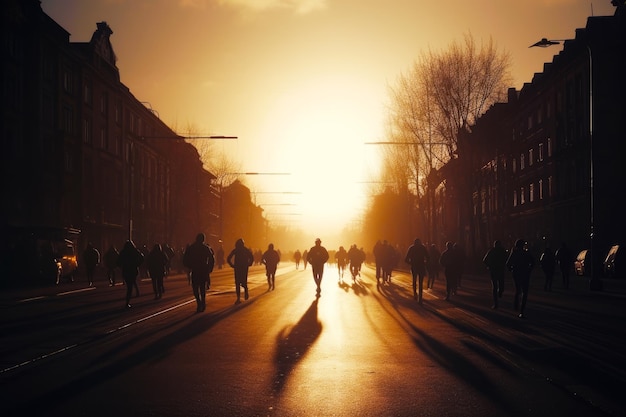In this evocative photograph, a bustling street is captured at sunrise, with the scene bathed in an intense, golden light. The brilliant sun dominates the sky, rendering the numerous pedestrians as dark silhouettes arrayed symmetrically down the street. Their indistinct forms stretch uniformly across the thoroughfare, creating an almost endless procession. A reflective sheen from the sunlight glistens on the concrete pavement, accentuating the street's lines and a faint center divider.

On both sides of the street, buildings stand tall. To the left, a structure with numerous windows—possibly a school—stands, its facade catching the early light. Adjacent to it rises another similar, though slightly taller, building. A lamppost is also visible on the left, though its light is off, overshadowed by the dawn’s splendor. Further in the background, taller trees loom, framing the urban landscape with a touch of nature.

The foreground is cast in deeper shadow, save for the distinct silhouette of a central figure. The interplay of light and shadow elongates this person's form, making them appear strikingly prominent against the backdrop. Their stance, either marching or fleeing, suggests a determined purpose or goal. The overall composition, punctuated by light and dark contrasts, evokes a narrative of motion and intent in the early hours of the day.